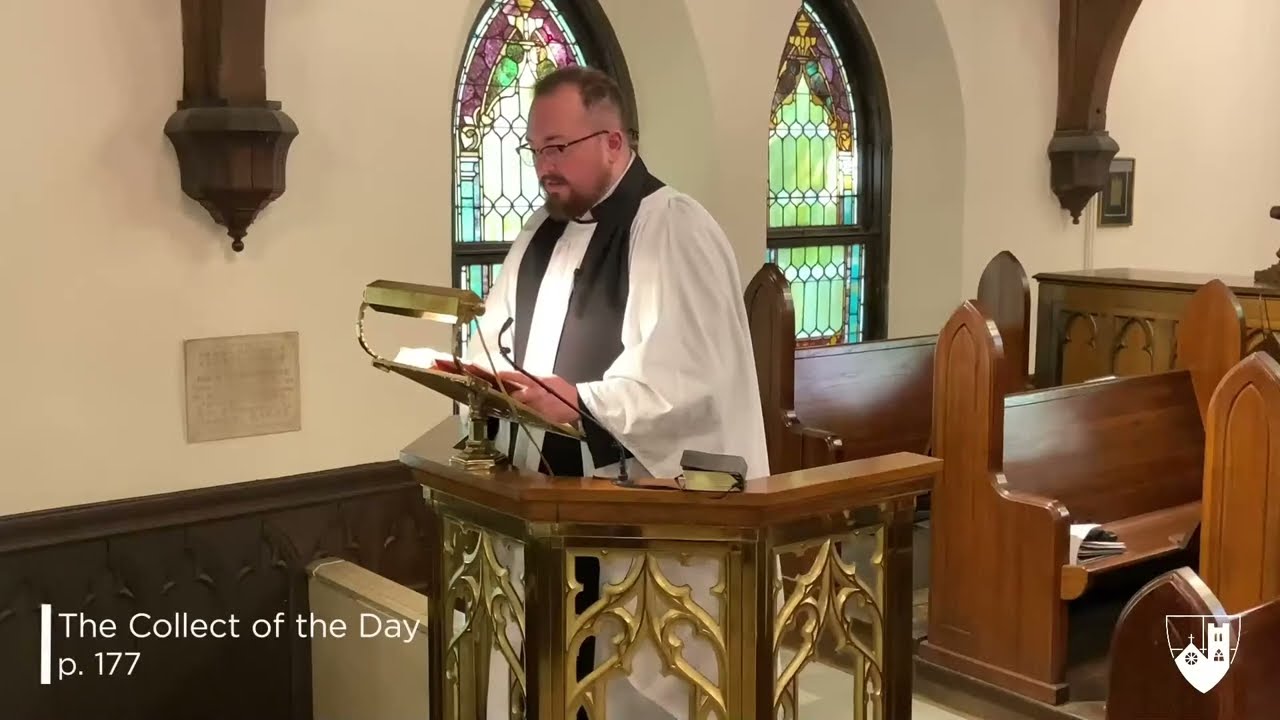In this image, a middle-aged priest, distinguished by his light skin and reddish-brown beard and mustache, stands solemnly at a lectern in a church. He is dressed in a long white robe with a black stole draped over his shoulders, lending him an air of traditional reverence. The priest wears black-framed glasses with clear lenses and is intently focused on the book in front of him, which is illuminated by a brass piano lamp attached to the intricately designed lectern. Inscribed on the lectern are the words "Collect of the Day, P.177," indicating a specific section of the liturgy. Behind him, the church’s rich brown wooden pews and cream-colored walls provide a warm backdrop, while arched stained glass windows, primarily tinted in green but varying in lighter shades due to the sunlight, add a touch of sacred artistry to the setting. The priest, likely delivering a sermon, stands alone with no other individuals visible, suggesting a moment of quiet contemplation or a service being recorded.